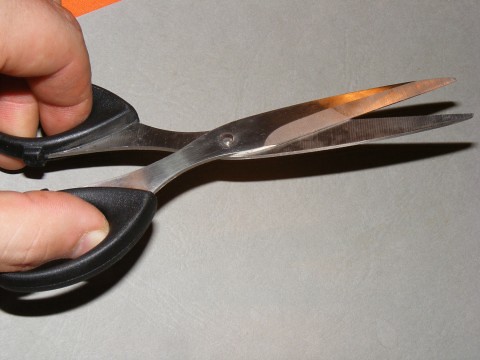In this close-up photograph, a pair of small, partially opened black-handled scissors are being held by a left hand, with the thumb, index, and middle fingers inserted into the scissor holes. The scissors, which are made of metal with a silver sheen, are positioned against a white background that resembles a piece of paper. The image shows the pronounced shadows of the scissors cast on this white surface. The surface itself appears to be placed on an orange area, visible in the top left corner of the image, casting an orange reflection on the shiny blades of the scissors. The person's hand is of lighter complexion, attributed to a European descent, and a reflection of an orange light on the metal of the scissors can be seen. The overall setting suggests a simple yet detailed arrangement, focusing on the interaction between the hand, scissors, and light reflections.